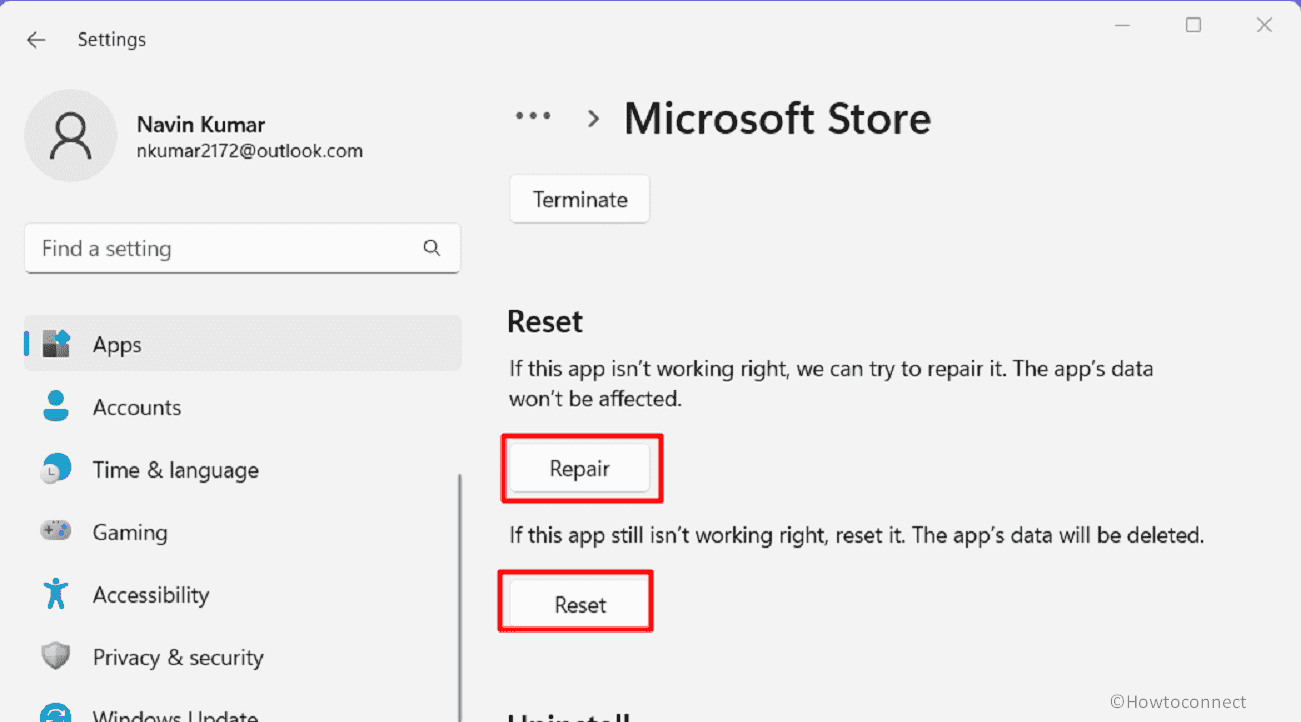This screenshot displays the settings interface of an application on a computer. In the upper left-hand corner, there is a circular gray silhouette icon accompanied by the name "Navin Kumar" and his email address. Nearby, an arrow points to the right with the label "Microsoft Store" and a "Terminate" option below it.

In the middle of the screen, the section titled "Reset" suggests troubleshooting steps for an app. It states: "If this app isn't working right, we can try to repair it. The app's data won't be affected," followed by a white "Repair" button outlined in red. Below, another message reads: "If this app still isn't working right, reset it. The app's data will be deleted," which is paired with a "Reset" button, similarly styled in a white rectangle with a red outline.

On the left-hand side, under the "Find a setting" section, there are icons representing different settings categories. These include:

1. Apps
2. Accounts
3. Time and Language
4. Gaming
5. Accessibility
6. Privacy and Security
7. Windows Update (partially visible and slightly cut off by the screenshot)

Each category is visually represented by its icon, denoting various configuration options available within the interface.